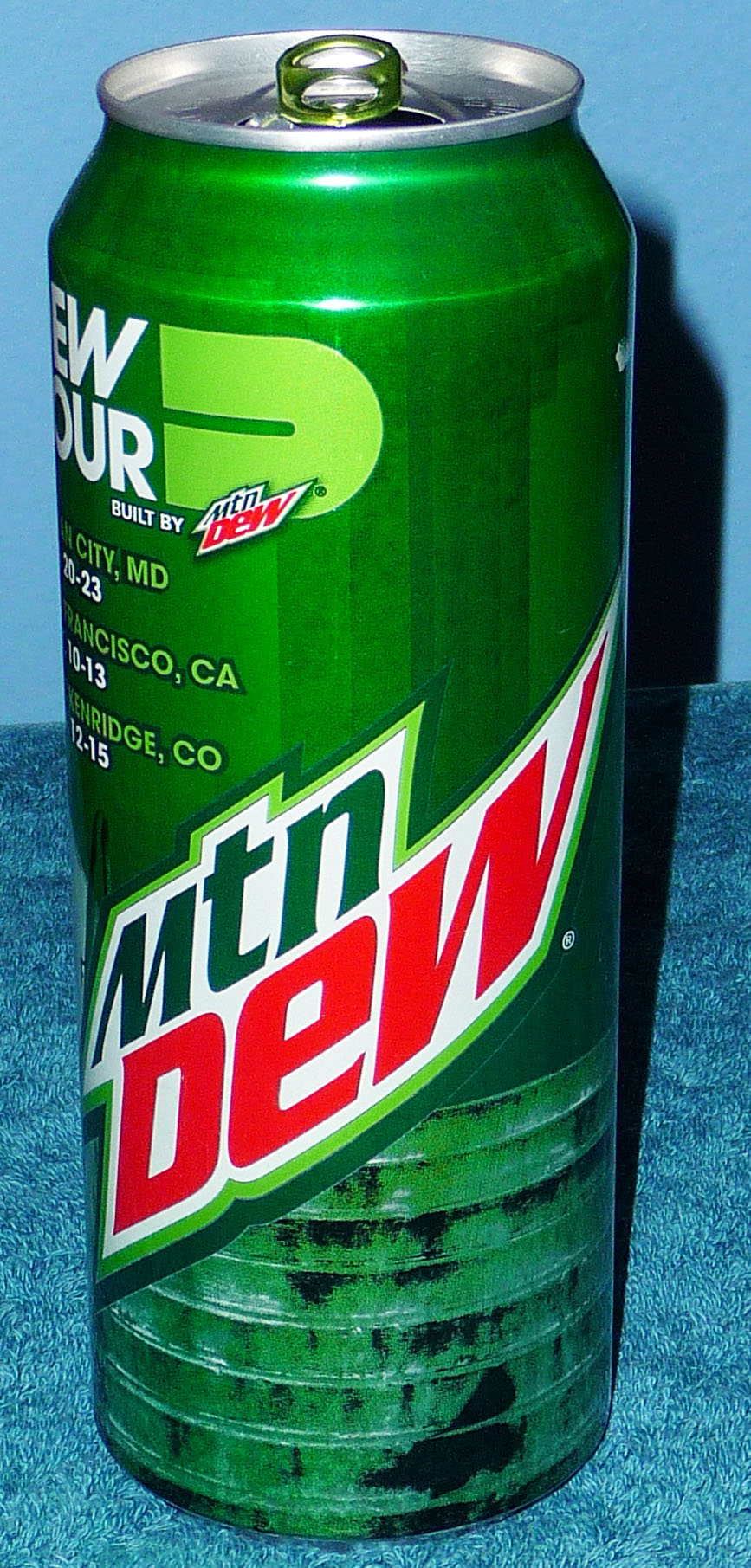This photograph, captured in portrait orientation, offers a close-up view of a can of Mountain Dew, a popular soft drink. Dominating the frame, the vibrant green can stands out against a background composed of a light blue wall and a deeper blue cloth surface that rises halfway through the photo. The top of the can is silver, featuring a raised pop top. The can's neck slightly narrows beneath the top before forming a solid cylindrical shape.

Central to the can's design is the Mountain Dew logo. Bold, dark green letters 'MTN' span diagonally from left to right, outlined in white for contrast. The iconic word 'DEW' appears below, rendered in larger red letters. Additional visible text near the top left includes partial white letters "E-W" and "O-R-U. Below this text, "Built by Mountain Dew" is written, signifying the brand's craftsmanship. Other informative lettering specifies cities like City, Maryland; Francisco, California; and Bridge, Colorado, displayed near the top left under the white script. Together, these elements create a visually striking and detailed portrayal of the Mountain Dew can.